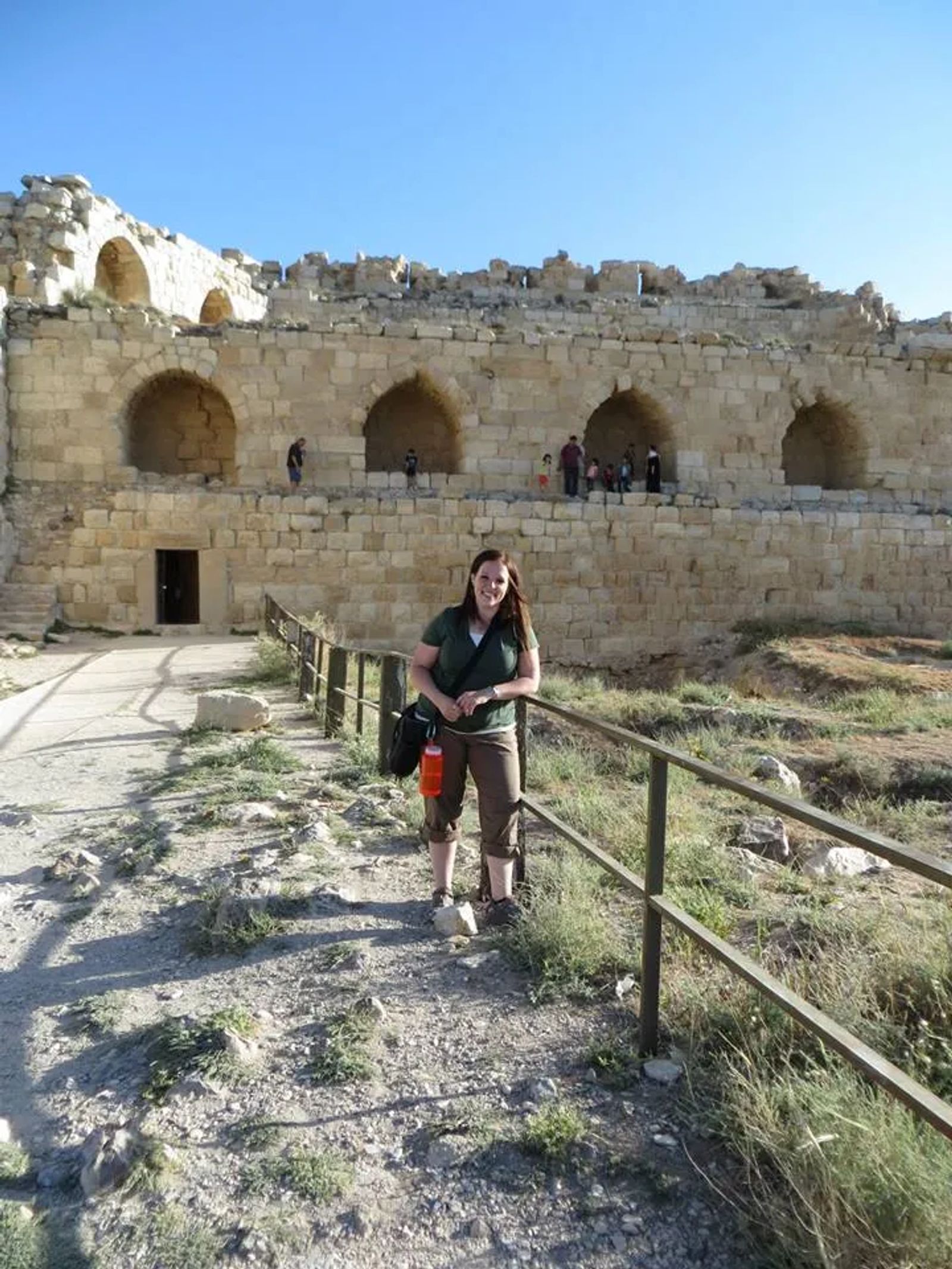This outdoor portrait photograph captures a woman leaned against a copper-colored metal fence on a rocky and dirt-covered walkway. The sunlit sky above is clear and a deep blue, unobstructed by clouds. Behind her stands a large, ancient stone structure, three levels high, constructed of tan-colored, cream stones. The second level features arched, open-air windows rather than glass panes, and the ground level has a single door, suggesting the building's historical significance and perhaps Middle Eastern origin. 

The foreground to the right of the woman reveals an overgrown area of unkempt grass and weeds. The woman, a Caucasian with brown hair, wears a green short-sleeved shirt, brown khaki pants, brown shoes, and carries a black purse along with a reddish-orange water bottle attached to her belt. She smiles directly at the camera, her arms comfortably clasped in front of her, adding a personal touch to the historic, rugged backdrop.